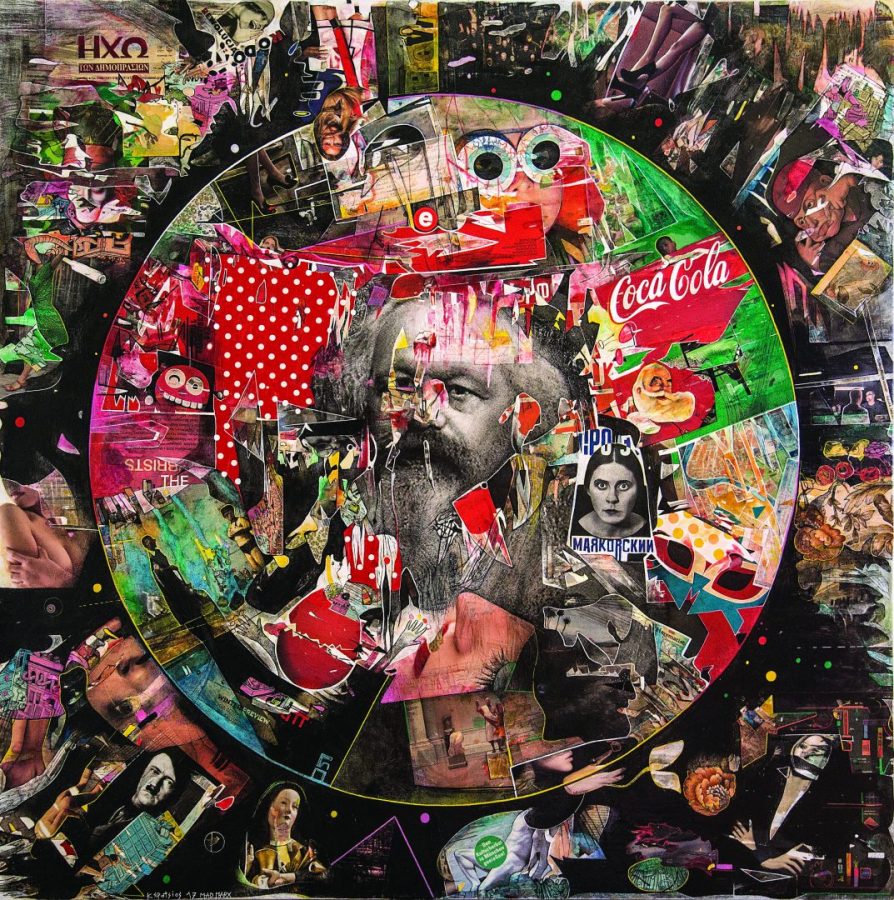The image is a highly detailed and busy collage that features a circular centerpiece brimming with an eclectic mix of pictures and icons. Dominating the center, there is an image of a bearded man, likely Karl Marx, surrounded by various other images, including a stunned-faced woman, large eyes, a child’s face, and numerous logos such as Coca-Cola and Marj Rickman. The central collage is infused with a red background patterned with white dots. Encircling this core, an even more chaotic array of images can be seen; these include historical figures like Adolf Hitler, artistic renderings, and possibly a Nutcracker or Lich performance. The background also features photographs of famous people, drawings, and photos that might depict adult content. The overall composition is overwhelming, with layers of visual elements densely packed together, making it challenging to distinguish each individual part.